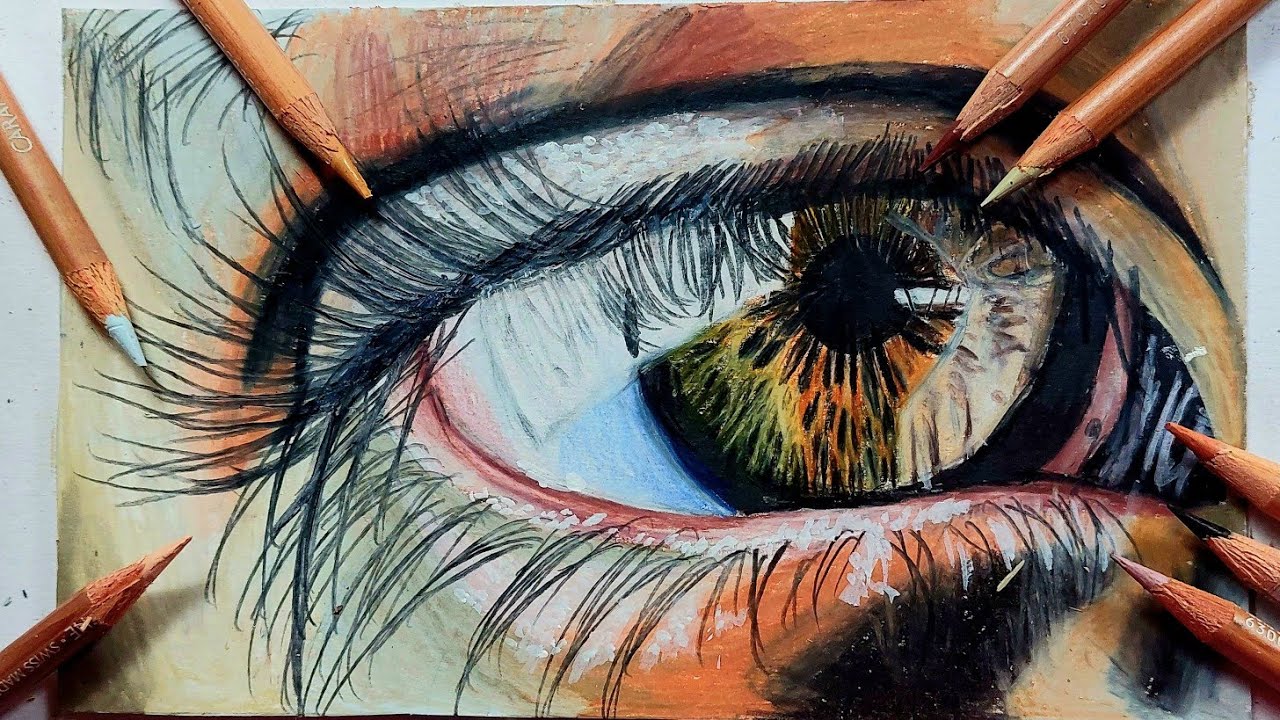This is a detailed illustration of a human eye, captured in a horizontal color photograph. The eye, filled with vibrant colors, has a pupil surrounded by hues of orange, yellow, green, blue, beige, and brown. The white part of the eye is tinged with blue. This striking eye features long, black eyelashes on both the upper and lower eyelids. The person's skin is a mix of orange and tan, with black shading resembling eyelashes in the background. Eight colored pencils, arranged deliberately around the drawing—five on the right and three on the left—indicate the tools used for this artwork. The pencils come in neutral skin tones, including whites, tans, browns, and black, complementing the colors within the eye. The entire image appears to rest on a white desk, though the close-up perspective focuses on the eye and pencils, excluding other elements.